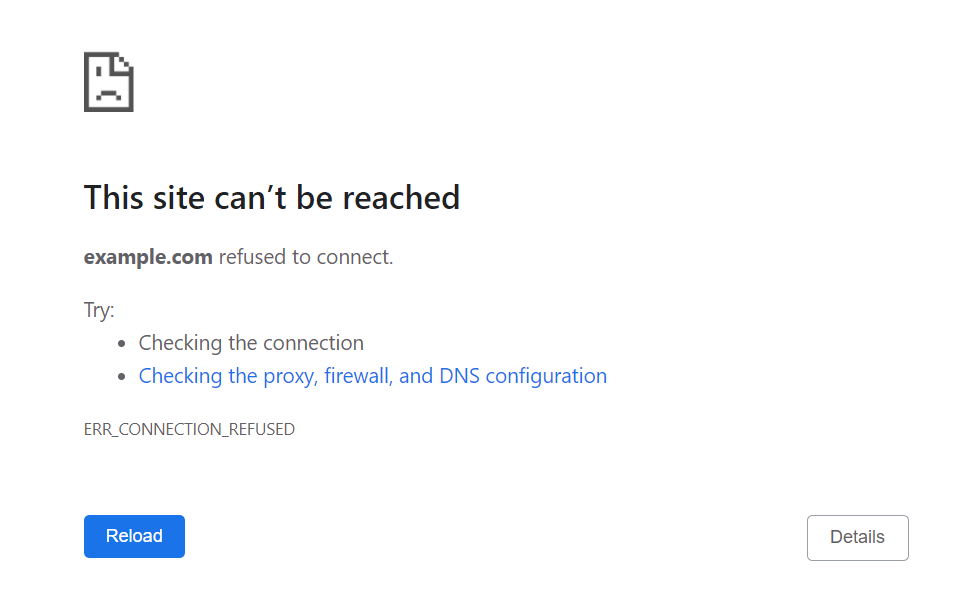An image showcasing a typical Windows error message with a clean, white background. Prominently displayed at the top is an icon depicting a page with a frowny face, a single visible eye, and a right-hand corner that appears cut off. Directly beneath this icon, in bold black text, is the message: "This site can’t be reached." Following this, in a lighter gray text, it states: "example.com refused to connect." Below this, further instructions in gray suggest actions to resolve the issue: "Try: - Checking the connection - Checking the proxy, firewall, and DNS configuration." At the very bottom of the message is an error code, "ERR_CONNECTION_REFUSED," rendered in gray. Completing the image, a prominent blue button labeled "Reload" in white text appears in the lower center area, while a smaller white button with gray text that reads "Details" is positioned in the bottom-right corner.